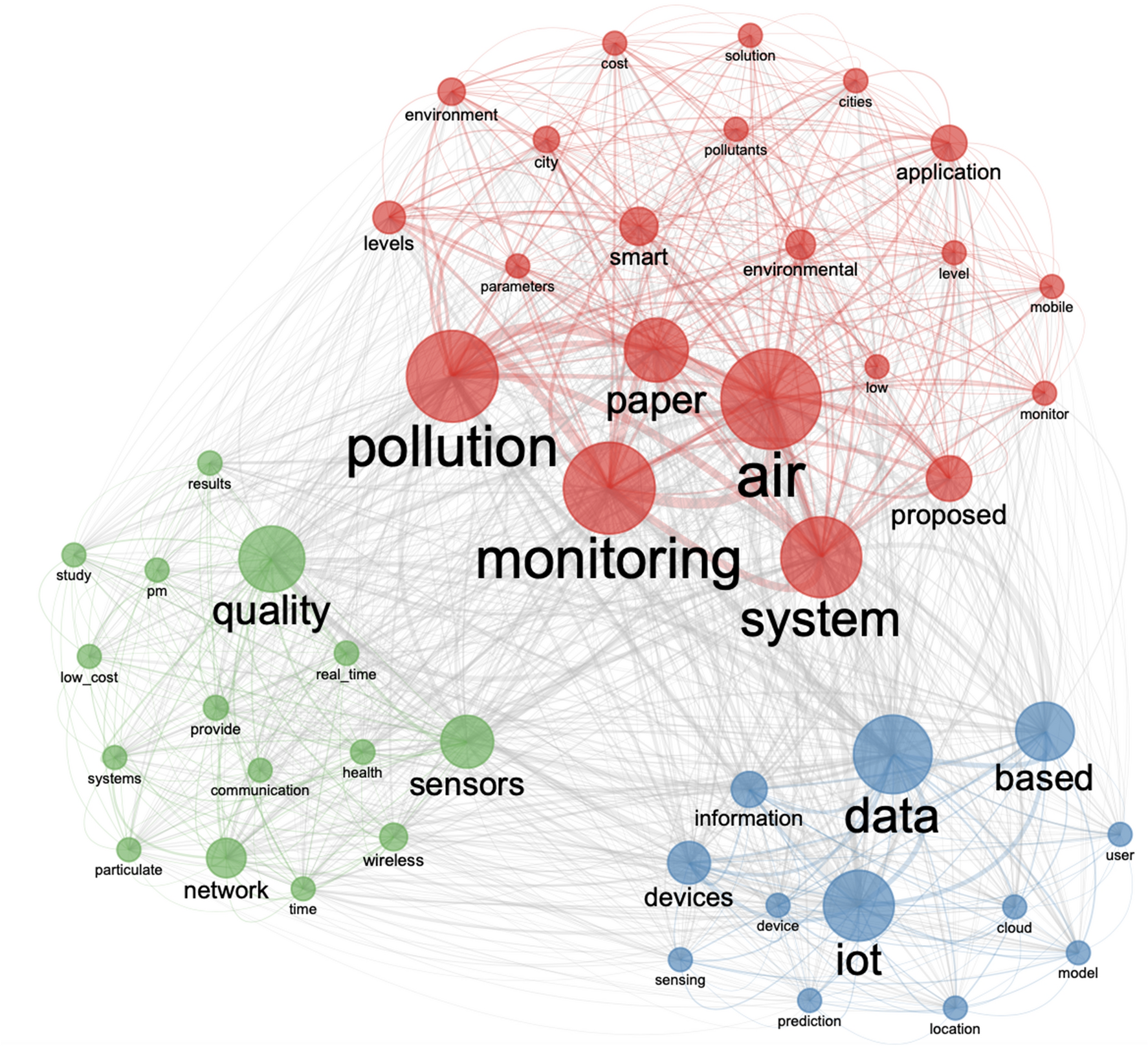The image displays a complex and detailed Venn diagram on a plain white background, divided into three main interconnected sections by colored circles and lines. In the upper right area, red dots dominate with larger ones labeled "Pollution," "Monitoring," "Air," "System," "Paper," and "Proposed," while smaller red dots label terms like "Parameters," "Levels," and "City." These red dots are connected by red lines, indicating their relationships.

In the lower left area, green dots represent terms related to air quality, with larger dots labeled "Quality" and "Sensors," and smaller ones labeled "Results," "PM," "Study," "Low Cost," and "Real-Time." These dots are connected by green lines, showcasing their interrelations.

In the lower right area, blue dots focus on data and technology, with larger ones labeled "Data," "IoT," and "Based." Smaller blue dots include terms like "User," "Model," "Cloud," "Location," "Prediction," "Device Sensing," and "Information." Blue lines connect these dots within the section.

Gray lines interconnect the three sections, visualizing the interplay between pollution monitoring, air quality, and data technology.